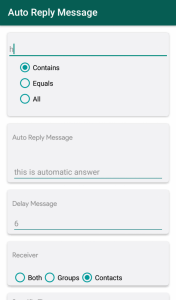The image displays a user interface for setting up auto-reply messages. The header, located at the top part of the image, features the title "Auto-Reply Messages" written in bold, black text. The background of the header is green, and the text is aligned to the top left corner. 

Below the header are sections for configuring the auto-reply messages. The first section is labeled "Text" and presents three options with circular checkboxes:

1. "Contains" (highlighted)
2. "Equals"
3. "All"

The second section is titled "Auto-Reply Messages." It includes a text input field labeled "This is an automatic answer," where the user can type the automatic reply message.

Following this, there is a section labeled "Delay Messages," accompanied by a numerical input field currently set to 6.

At the bottom of the image, the "Receiver" section offers three options for selecting recipients of the auto-reply messages:

1. Both Groups and Contacts
2. Contact (highlighted in green)

The text throughout the interface is written in black, whereas interactive elements like checkboxes and input fields have a green or light green color scheme. The checkboxes are circular rather than square.